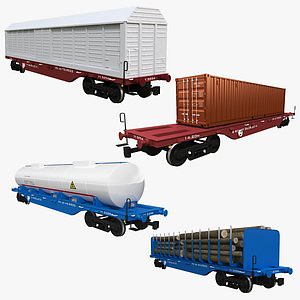This color photograph features a detailed display of four different trailer compartments, all mounted on black 18-wheel frames. In the top-left corner, there is a white trailer with a red base, resembling a covered shipping container with a gable roof structure. Below it, to the right, is another trailer with the same red base and black tires, but this one has a red-orange compartment, indicating it's a common shipping compartment. In the bottom left, you can see a blue-based trailer supporting a large white cylindrical tank, clearly designed as a fuel tanker. Finally, in the bottom right, there is a fully blue trailer, which is an open flatbed loaded with lumber.